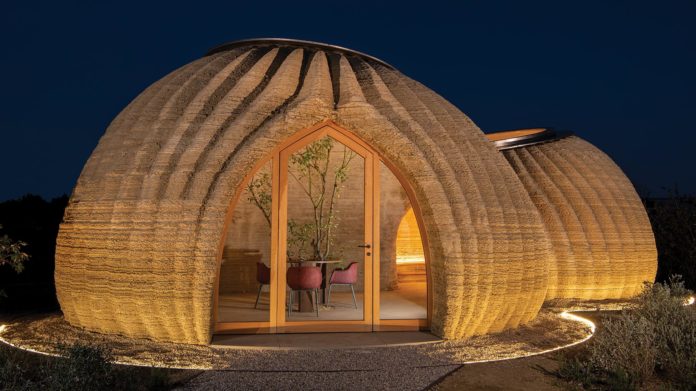The photograph is a full-color, nighttime outdoor scene with a horizontally rectangular format. The dark sky in the background has a faint bluish tint, though it lacks visible stars. On both the lower left and right corners and also towards the center left and center right, patches of vegetation are discernible, adding some natural elements to the scene.

The primary focus of the image is a pair of uniquely designed buildings that resemble onion-shaped or beehive-like structures. These buildings feature a distinct vertical texture that runs from their base to the top, accentuating their rounded, pod-like appearance. The buildings are tan and appear to function as enclosed patio spaces.

Central to the image is an archway that includes a framed glass door. The door's design is notable, incorporating glass panels and having a shape that resembles a square topped with a triangle. Flanking the doorway on either side are two sidelights that help illuminate the entrance. Through the glass door, the interior is visible, showing a table, three red chairs, and what appears to be a tree growing up from the table, creating an intriguing visual focus.

In addition to this, there are black bars extending from the top of the buildings, and various lights are visible, giving the structures a connected, resort-like ambiance. The overall scene conveys a whimsical, almost surreal atmosphere with these illuminated, futuristic pods set against a serene, dark nighttime backdrop.